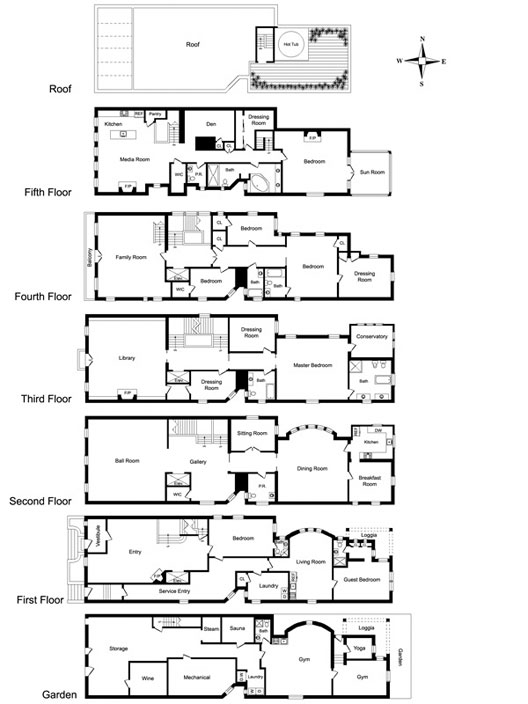The image displays a detailed blueprint set against a white background. In the top right corner, there is a compass rose, a small four-pointed star indicating north, south, east, and west. At the top of the blueprint, the roof plan is depicted, showing a small square protrusion, likely an air conditioning unit. 

The blueprint then delineates the fifth floor, which outlines various rooms in black with light gray lines detailing the interior structures. Moving to the fourth floor, the layout includes a large main area that appears to be a family room, a small bedroom, and a dining room. The third floor features a spacious living room, another dining room, a master bedroom, and a bath. The second floor comprises another bedroom and a dining room, while the first floor includes an entryway, several other rooms, and an adjacent garden area.